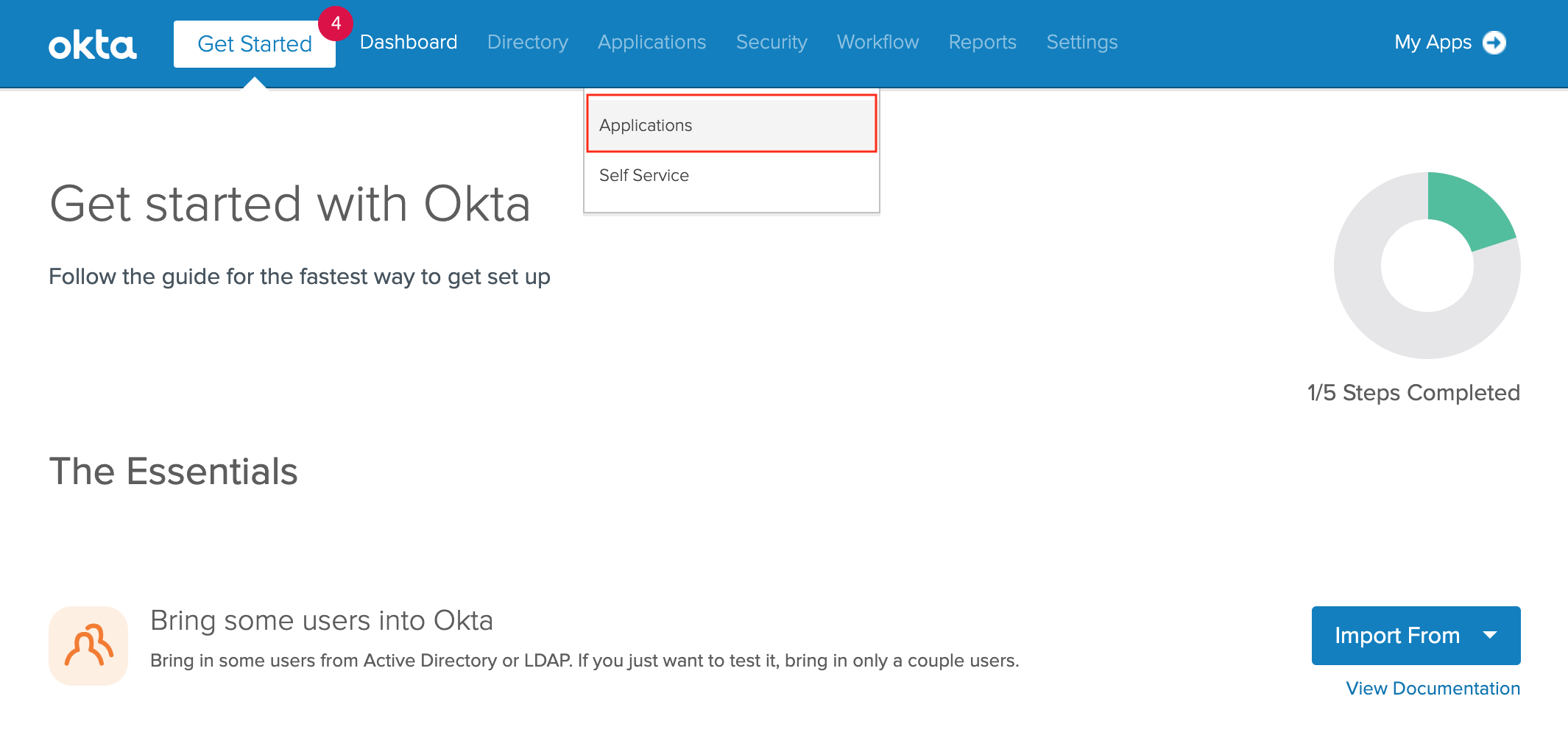This image is a screenshot from the Okta website, which is an identity and access management platform. At the top left corner of the image, "okta" is written in lowercase letters within a long, skinny blue rectangle. Adjacent to this, on the blue bar, there is a white box labeled "Get Started," highlighted by a white number four inside a red circle, reminiscent of a notification badge.

Following this, a navigation menu lists several options: Dashboard, Directory, Applications, Security, Workflow, Reports, and Settings. At the far-right end of the blue rectangle, the text "My Apps" is accompanied by a rightward-pointing arrow. Below this navigation bar, a donut-shaped gray circle displays progress, with the center in white and a green segment indicating that 1 out of 5 steps have been completed.

In the central area of the image, framed by a red rectangular outline, is the "Applications" section. Within this frame, the text encourages users to "Get started with Okta" and follow a guide for the quickest setup. There are sections titled "The Essentials" and "Bring Some Users into Okta."